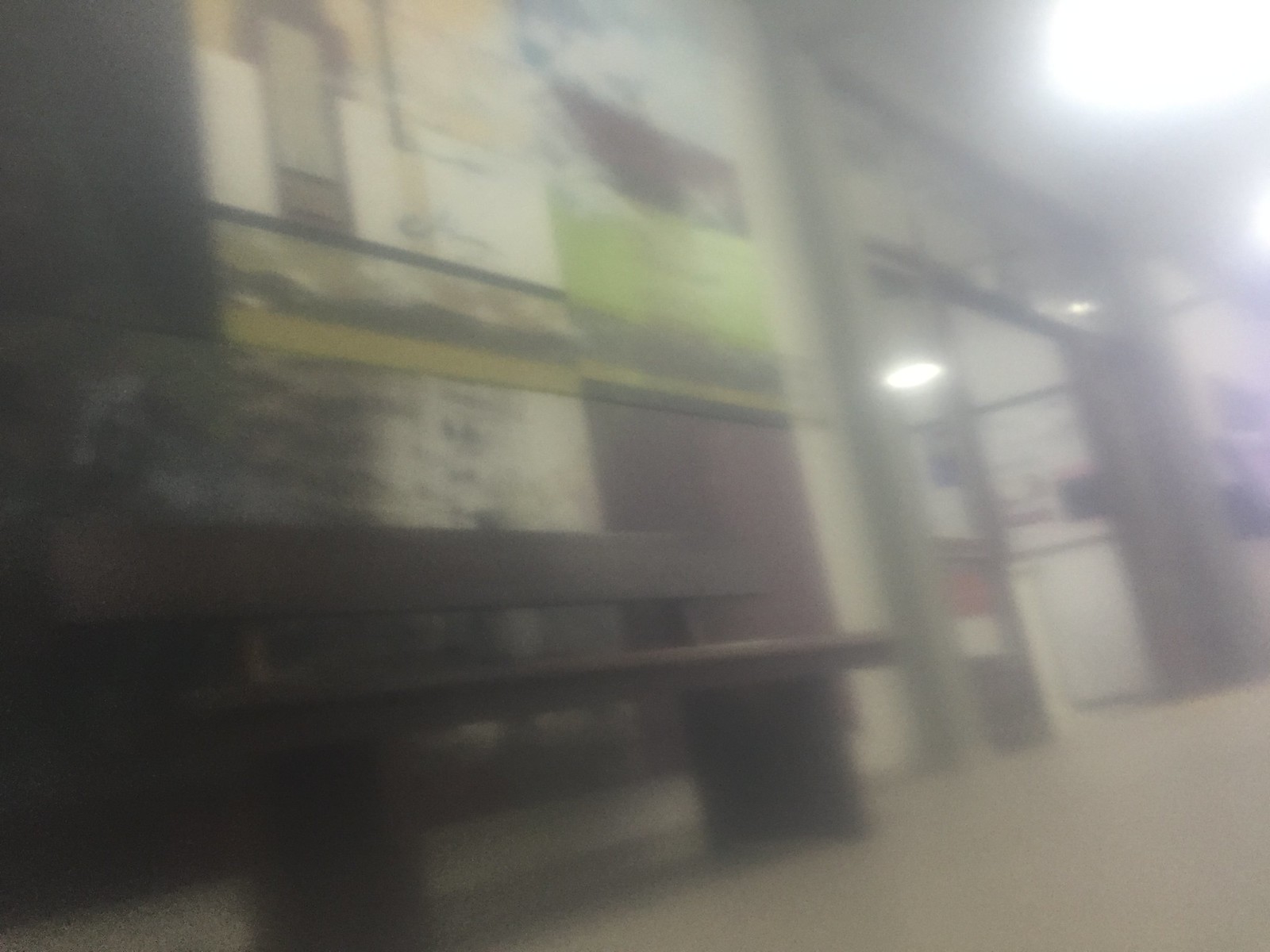This photograph, though significantly out of focus, captures an indoor scene viewed from a downward-tilting angle to the left. In the foreground, a brown bench with a backrest is prominently visible. To the right of the bench, a doorway likely leads into a store. Behind the bench, the wall is adorned with several posters that have a commercial appearance, adding to the indoor ambiance. The top portion of the image is dominated by intensely bright lights, which contribute to the blurriness and cause the details in this area to fade out, further obscuring the scene.